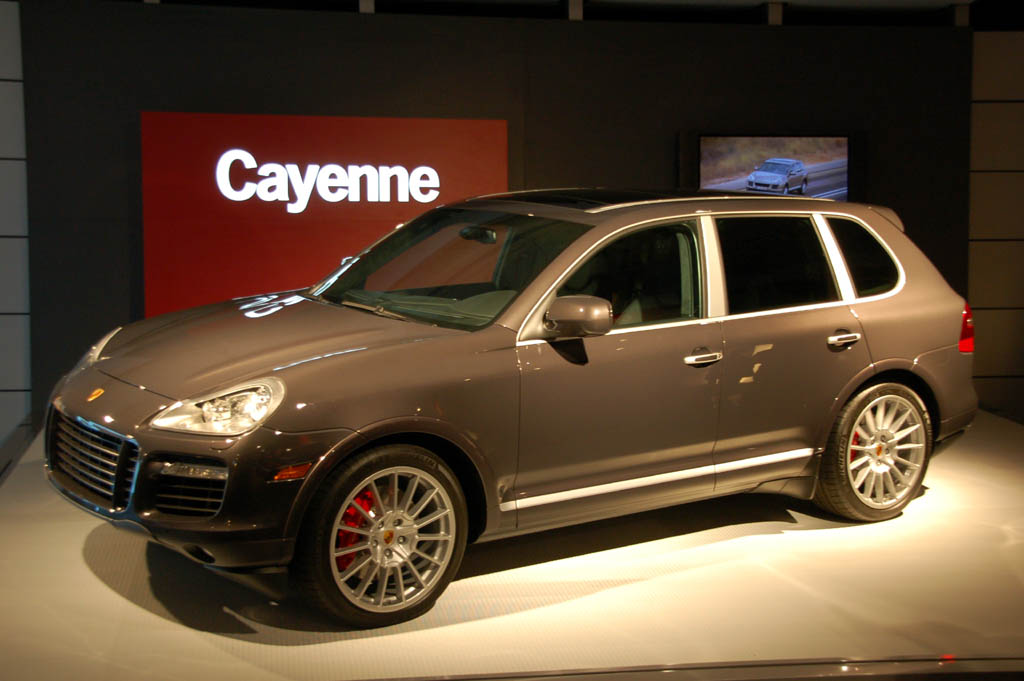The image displays a dark grey Porsche Cayenne SUV showcased in a car dealership showroom setting. The showroom floor is made of light colored, grey or white tiles, contrasting with the darker backdrop. The back wall, framed with white tiles, features a large red square panel with white text displaying the word "Cayenne" on the left side. To the right, a small television screen shows a video or image of the Cayenne driving along a roadway. The car is brightly lit, sitting on metallic silver and black-rimmed wheels, and boasts striking white front headlights. The entire scene is devoid of people, allowing the focus to remain solely on the polished, slightly reflective vehicle.